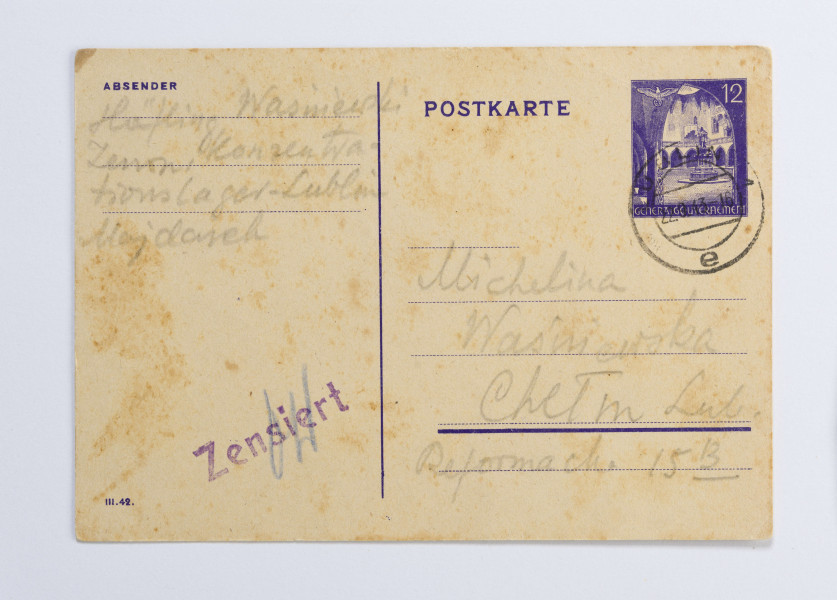The image depicts the back of an aged, beige postcard speckled with brown spots and stains, giving it a dirty appearance. The postcard features primarily purple ink, including a distinct stamp at the top right, depicting a Nazi eagle and the number "12." The word "POSTKARTE" is clearly printed in purple on the upper right side. Adjacent to this are purple lines for writing, filled with very faint, almost invisible gray pencil markings, possibly in German. On the left side of the postcard, there's a purple stamp angled diagonally that reads "ZENSIERT," with blue initials superimposed on it. At the top left corner, "AB SENDER" is printed, accompanied by faded handwriting.